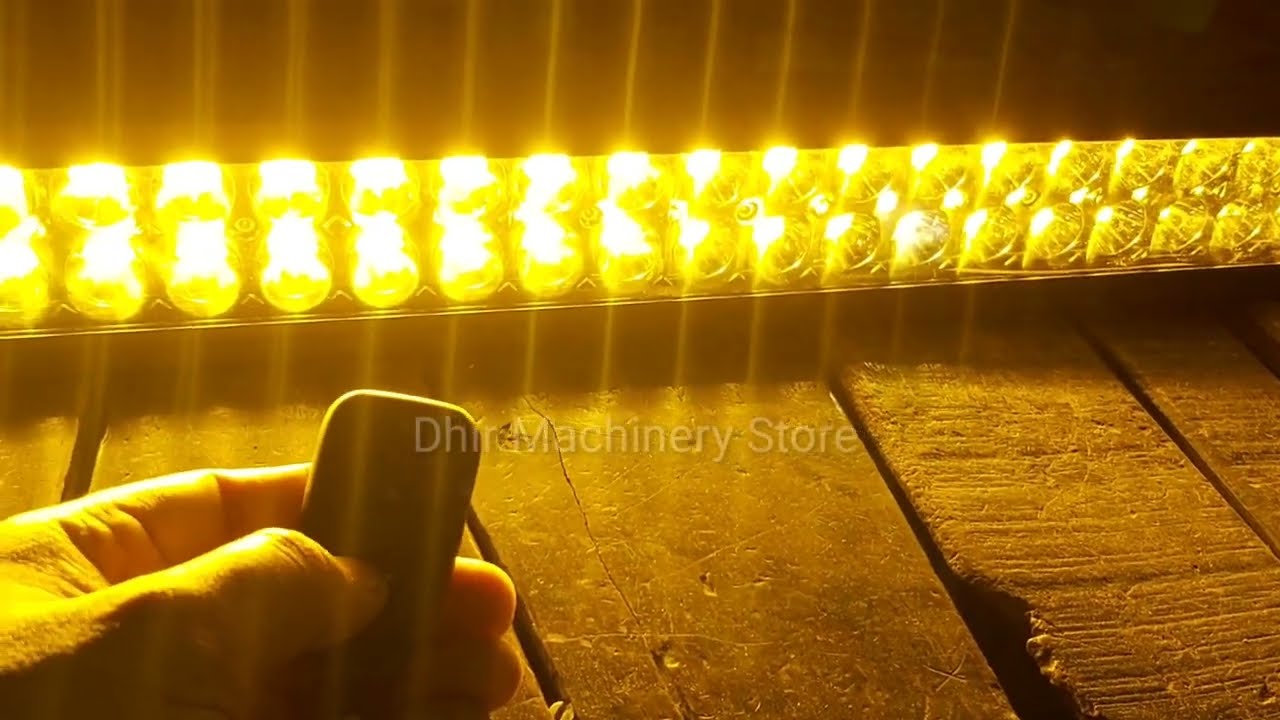The image captures a nighttime outdoor scene featuring several distinct elements. At the bottom of the frame, there is a worn, potentially cracked wooden surface, which could be either a table or a floor. Dominating the bottom left corner, a man's hand is seen holding a black remote or switch with his thumb pressing a button. The top section of the image is defined by a horizontal stripe of bright yellow lights stretching from left to right, casting white shadows and forming vertical yellow lines that suggest the edges of a rectangle. The background appears mostly black, emphasizing the stark contrast of the illuminated area. Additionally, a faint watermark reading "DHIR Machinery Store" is visible in the center of the image, hinting at the potential context or source of the scene depicted. The overall lighting and positioning suggest someone is in the process of operating or turning on the lights, with the diverse hues of black, white, yellow, gold, and brown contributing to the visual composition.